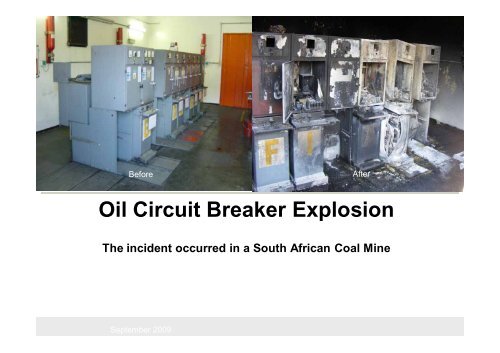This image captures a stark before-and-after sequence of an oil circuit breaker explosion in a South African coal mine, documented in September 2009. The lower half of the image is captioned with "oil circuit breaker explosion" in black text on a white background, accompanied by a light gray bar at the bottom bearing the same words in white text along with the date. 

The top part of the image is split into two photos. The left photo, labeled "before," features a row of large gray metal boxes, which are oil circuit breakers, situated in a white room with a red (or possibly orange) door in the background. The room is equipped with fire extinguishers on the walls, and a black box, potentially a vent, is visible. The oil circuit breakers appear to be unblemished and orderly, extending from the foreground to the background, indicating there might be around six to fifteen of these devices.

The right photo, labeled "after," provides a close-up view of the same oil circuit breakers post-explosion. The devices, previously gray, are now extensively damaged, with visible burns turning parts of them black and white. Panels have blown off, fallen apart, and lie scattered on the floor. Most of the upper-tier circuit breakers have exploded, sparing only a couple of units on the bottom tier. The metal boxes display significant discoloration and debris, vividly illustrating the aftermath of the devastating explosion.